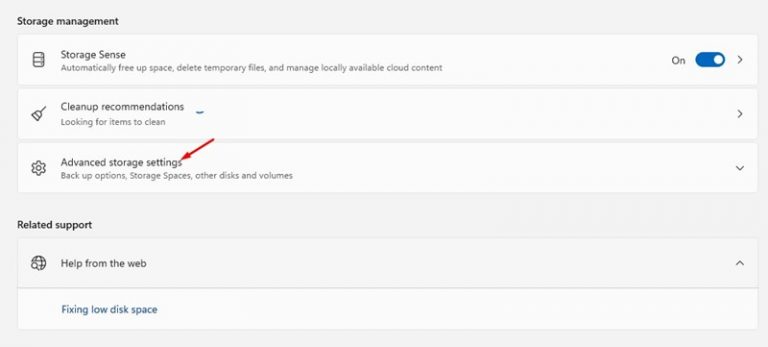### Websites

#### Storage Management Interface

This section provides a concise overview of the storage management features available on the website. It is framed by a grey border and segmented into distinct areas for easy navigation.

**Heading:**
- The top bar, set against a grey background, prominently displays "Storage Management" in bold, black letters.

**Main Section:**
- **Storage Sense:**
  - A white box contains text detailing the functionality of Storage Sense: "Automatically free up space, delete temporary files, and manage locally available cloud content."
  - A blue toggle switch indicates that Storage Sense is activated.
  - A right-facing arrow is present, allowing users to expand for more information or to navigate to that section.

- **Cleanup Recommendations:**
  - This section is actively searching for items that can be cleaned.
  - An icon of a broom is next to the text, signifying the cleaning action.
  - Like Storage Sense, it also features a right-facing arrow for additional options.

**Settings and Advanced Options:**
- At the lower portion of the main section, the gear icon signifies settings.
- Underneath, it mentions "Advanced Storage Settings," highlighted with a red arrow pointing to it, leading to further options such as Backup Options, Storage Spaces, and Other Disks and Volumes.

**Related Support:**
- Below, there is a smaller grey area with black text labeled "Related Support."
- This section includes a World Wide Web icon followed by "Help from the Web."
- A link in blue letters reads "Fixing Disk Space," offering users external help content.

In summary, this detailed caption depicts an image of a storage management interface, describing the layout, key functionalities, settings, and support options available to users.